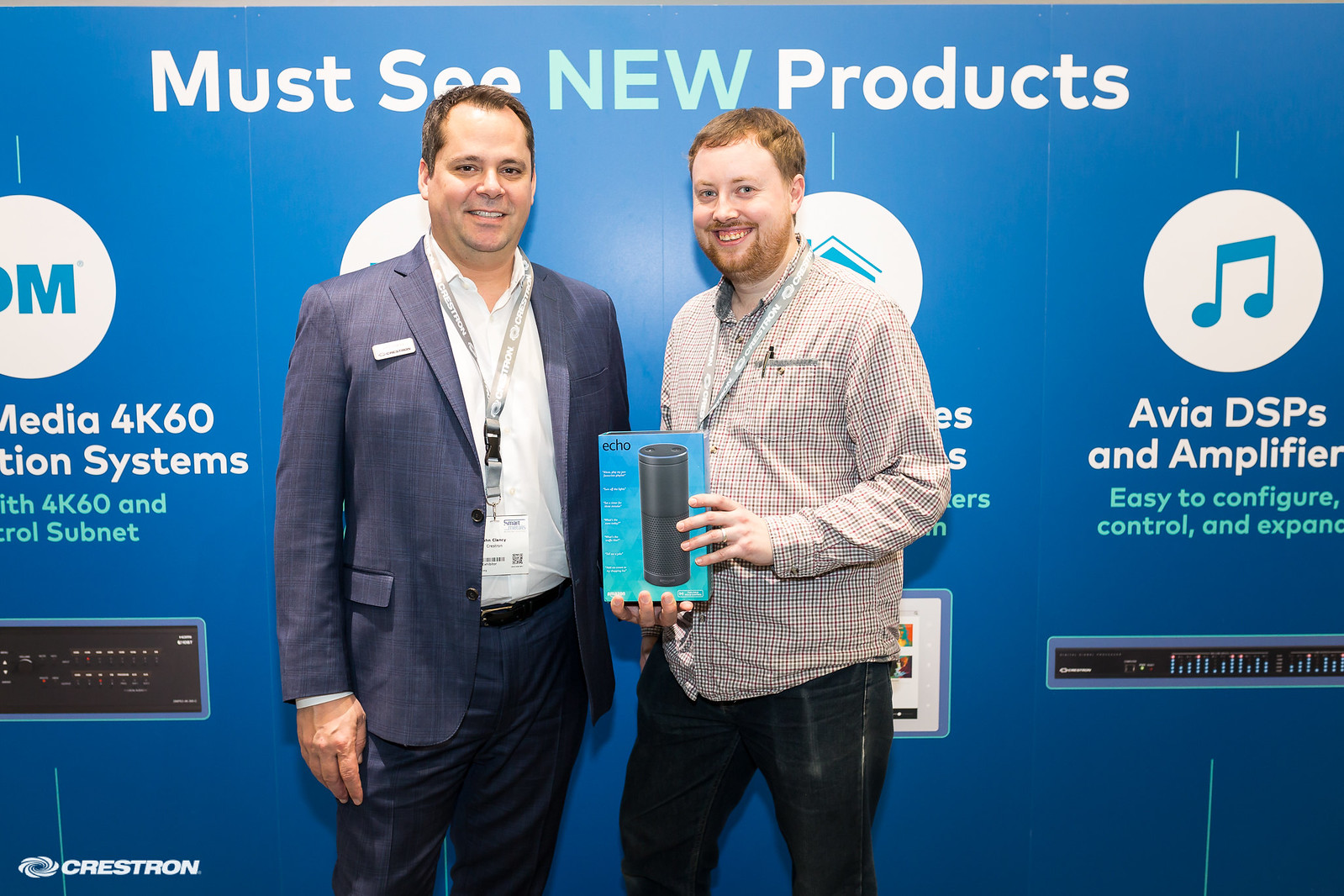This detailed photograph captures two men standing on a stage at an AV (Audio-Visual) conference. They are presenting new products in front of a blue wall adorned with the prominently displayed white text, "Must See New Products," with the word "new" highlighted in a light blue or green color. Below this headline, the wall features white circles with images, including a letter 'M' and a blue music note icon. Additional text on the wall describes the offerings: "Media 4K 60-something Systems" and "AVIA DSPS and Amplifiers," followed by the phrase, "Easy to configure, control, and expand."

The man on the left is wearing a dark blue suit with a white shirt, open collar, and no tie. He has brownish-red hair. The man to the right is casually dressed in blue jeans and an untucked, long-sleeved pinstripe shirt. He has red hair, a beard, and is holding a boxed product resembling a Bluetooth speaker labeled "Echo," likely an Amazon device. Both men appear to be demonstrating or promoting the company's latest developments in AV technology. The image is rectangular, wider than it is tall, and includes a narrow white header at the top, emphasizing the professional and modern setting of the conference.